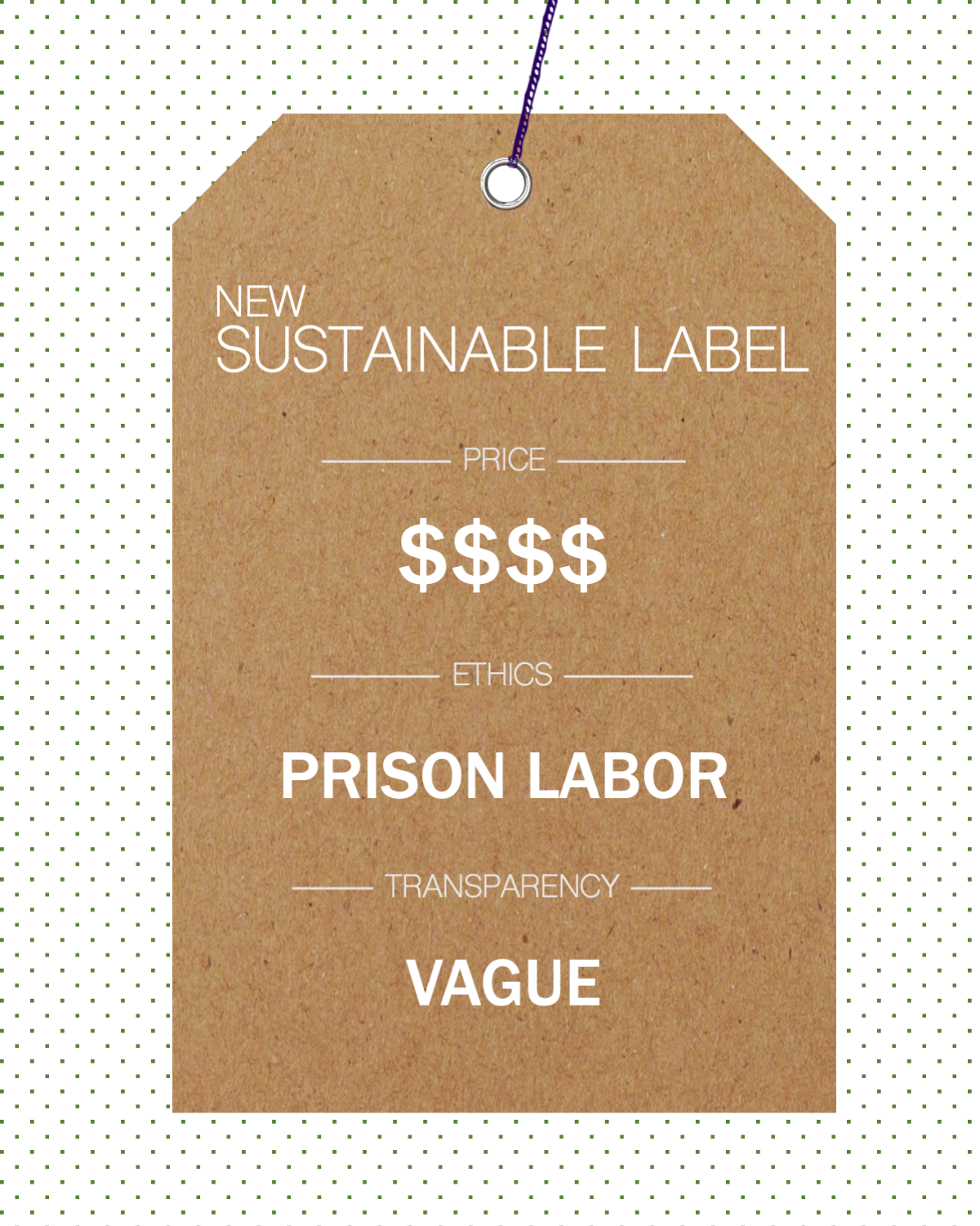This is a detailed close-up photo of a hexagonal kraft paper sales tag, light brown in color, with a silver grommet at the top center. Threaded through the grommet is a purple-blue string. The tag is set against a black-and-white polka dot background, laid out in a gingham pattern. The text on the label, all in white font, reads "NEW SUSTAINABLE LABEL" at the top, followed by "PRICE:" and four dollar signs ($$$$) indicating a place for the price. Below this, the label includes the white-printed words "ETHICS" with a horizontal line on either side, "PRISON LABOR" in bold capital letters, "TRANSPARENCY" also with lines on either side, and ending with "VAGUE" in bold capital letters. The label appears to be a parody, critiquing the ambiguity of ethical claims on products.